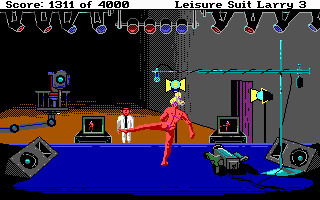In this pixel art image resembling a still from a video game, the scene is set on a stage under the title "Leisure Suit Larry 3." At the very top of the image, a status bar displays, "Score: 1311 of 4000." On stage stands a naked figure with orange skin, viewed from the back. The stage is illuminated by overhead spotlights in various colors—some red, some blue, though they are currently unlit. 

A microphone on a boom stand is positioned near the figure, flanked by two large speakers. The stage floor is a vibrant blue. In the background, where the audience would presumably be, are two monitors. One screen mirrors the figure’s pose exactly, while the other displays his leg in a different pose. 

Also present is a man adorned in a white shirt, light-colored pants, and a dark tie, with similarly orange skin. He appears to be involved in recording the scene, as there is a peculiar-looking camera on a boom pointed towards the stage. This entire setup is located within a vast, cavernous space. The orange figure on stage is striking a dynamic pose with his left leg stretched out to the side and his right arm extended for balance.